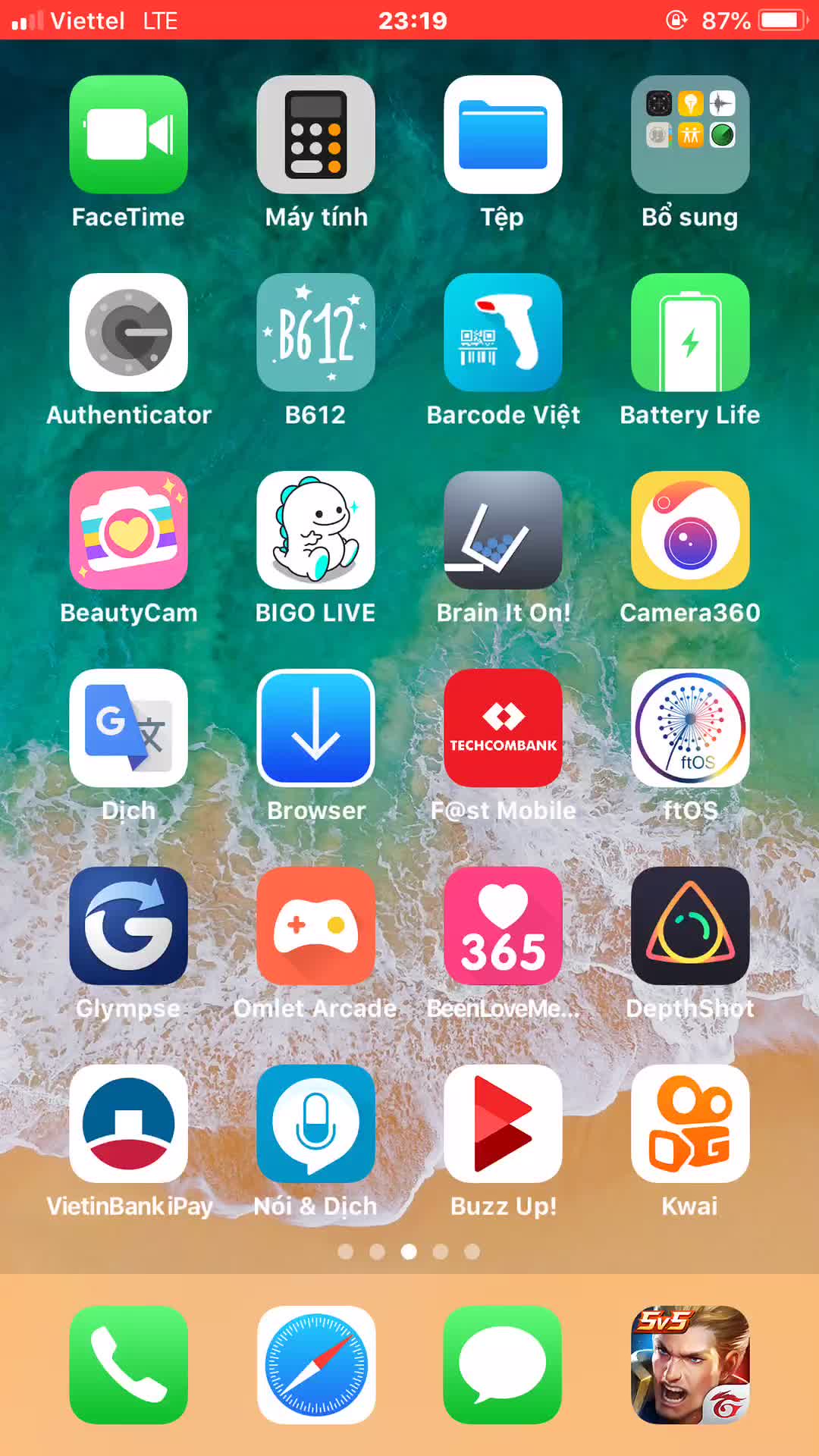The image depicts the home screen of a smartphone, featuring a serene background image of a sandy shore. The backdrop showcases aquamarine water and the white foam of gentle waves washing over the sand. The home screen is populated with several app icons, arranged in a structured grid of four columns extending from the top to the bottom of the display. These app icons come in a variety of colors, including green, blue, pink, orange, and red, adding a vibrant touch to the scene.

At the top of the screen, a red indicator bar is prominently visible. Positioned to the left side of this bar is the network name, Viettel LTE, signifying the carrier. Centrally placed within the red frame is the current time, displayed as 23:19 (11:19 PM). On the right side of the indicator bar, the battery level is shown, indicating a remaining charge of 87%. This meticulously detailed layout merges functionality with the tranquility of the seaside background, making for a visually appealing home screen.